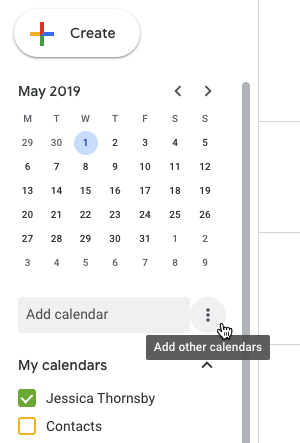The image depicts an interface of Google Calendar from May 2019. On the left side of the screen, there is a pane featuring a monthly calendar view with May 1st, a Wednesday, specifically highlighted. Below the calendar, under the section labeled "My Calendars," two calendar options are listed: "Jessica Thornsby," which is checked, and "Contacts," which remains unchecked. At the top of this pane, a large "Create" button is visible, suggesting the functionality to add a new event.

Hovering over the calendar interface is a cursor positioned near a text field labeled "Add calendar," accompanied by additional options to the right under "Add other calendars." This implies the ability to integrate events from various calendars into one view. The right side of the image features additional elements which appear to belong to the same or another scheduling tool, potentially indicating a schedule planner or agenda, giving the impression of a calendar within a calendar for comprehensive event management.